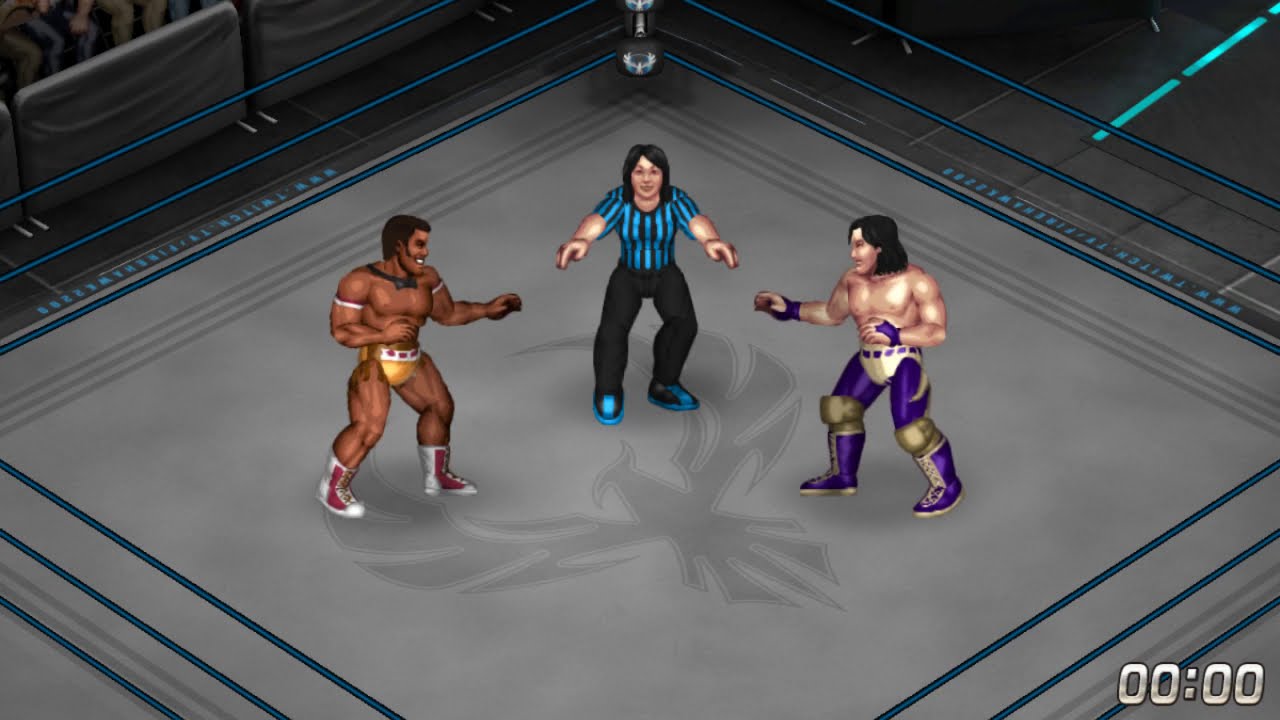The image is a detailed screenshot from a fighting video game depicting a wrestling match. In the center of a square wrestling ring with dark gray matting bordered by elastic ropes, a referee dressed in a blue-striped shirt and black pants has his arms outstretched, signaling the start of the fight. Dominating the ring's center is an emblematic phoenix symbol. On the left side of the ring stands an African-American wrestler, and on the right is a light-skinned Asian wrestler, both adorned in gaudy pro wrestling attire, with one wearing wrestling trunks and boots and the other in pants without a shirt. The stylized, cartoonish art further indicates that this is part of a video game, possibly "Fire Pro Wrestling." Visible colors in the scene include brown, gold, white, red, blue, purple, gray, and black. Notably, a timer in the bottom right corner of the screen reads "00:00," indicating the fight is about to begin.